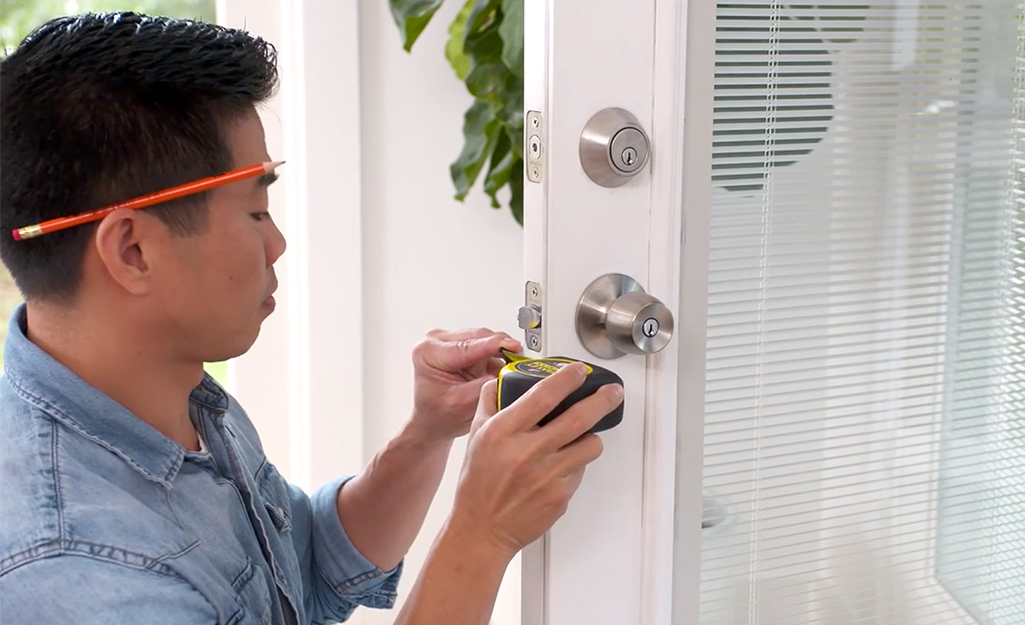This photograph features a side profile of an Asian male, likely in his early thirties, with short, black, gelled hair. He is meticulously measuring the width of a white door with a silver chrome handle and lock using a yellow and black tape measure. The man is wearing a faded blue denim shirt with its sleeves rolled up halfway. Notably, a large red pencil is propped up behind his right ear. His focused gaze is directed at the measuring tape, which is positioned just below the door's lock. The door he is measuring has a window fitted with small Venetian blinds. In the background, white walls are visible, as well as large leaves from a substantial plant. The man appears to be either kneeling or squatting, as his face is roughly at the height of the door handle while he partially opens the door during the measurement.